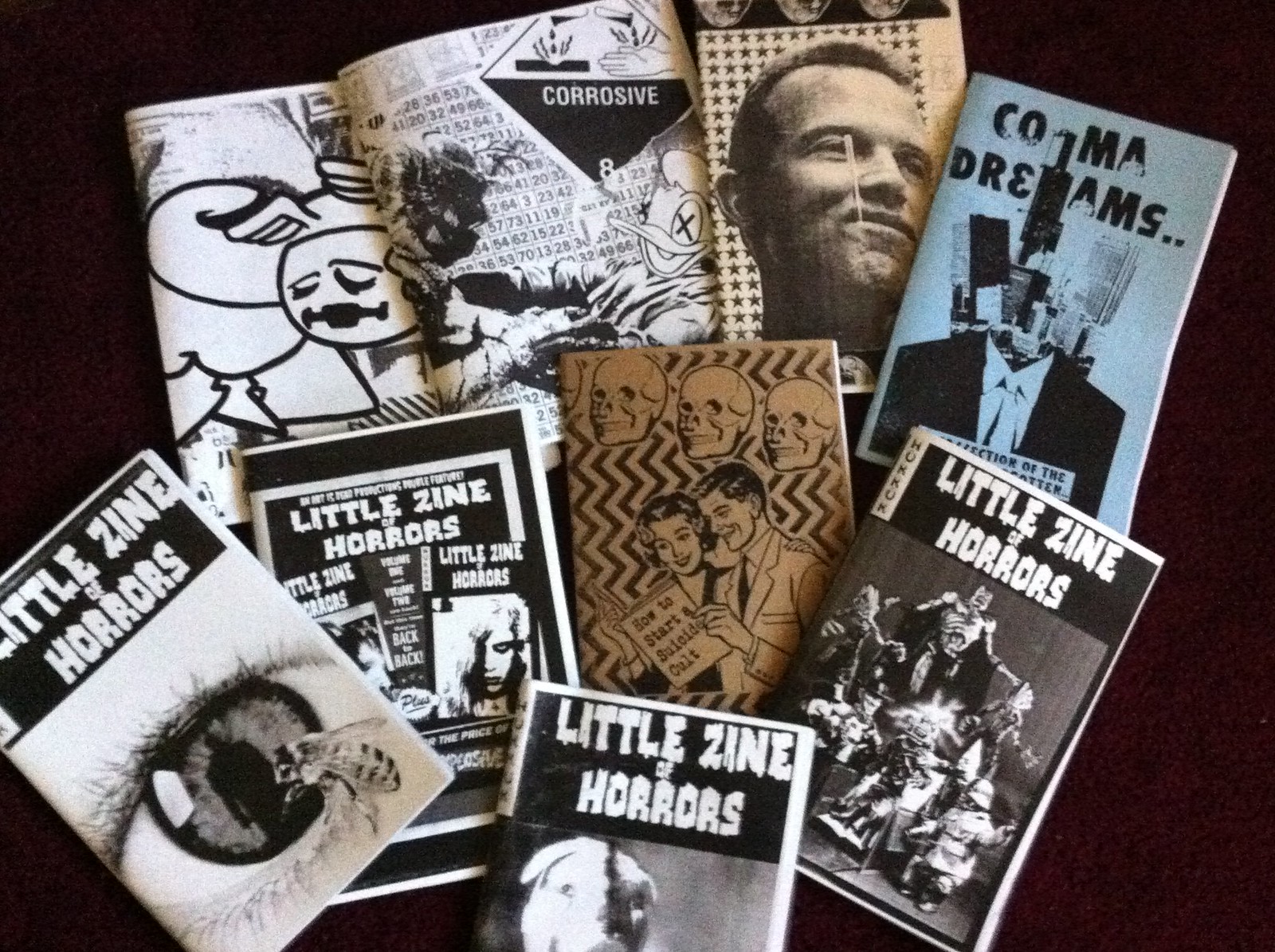This photo captures a collection of vintage horror magazines displayed against a dark maroon background, which could be a blanket or carpet. The focal point is a variety of small magazines, mostly titled "Little Zine of Horrors," with around eight issues spread out. The magazines predominantly feature black and white covers with eerie and unsettling visuals, characteristic of the horror theme. 

One cover on the left is primarily white and showcases a close-up of an eye, reflecting a person in dark attire, with a honeybee approaching it. Another magazine features a light-skinned man with dark hair. The central magazine has a striking black and white vertical zigzag design with three skulls at the top and a 1950s-style sketched man and woman, both smiling as they read a pamphlet titled "How to Start a Suicide Cult." Additionally, there's a magazine titled "Coma Dreams." Overall, the images range from horror elements like skeletons, monsters, and skulls to bizarre and creepy art, reinforcing the macabre theme of the collection.